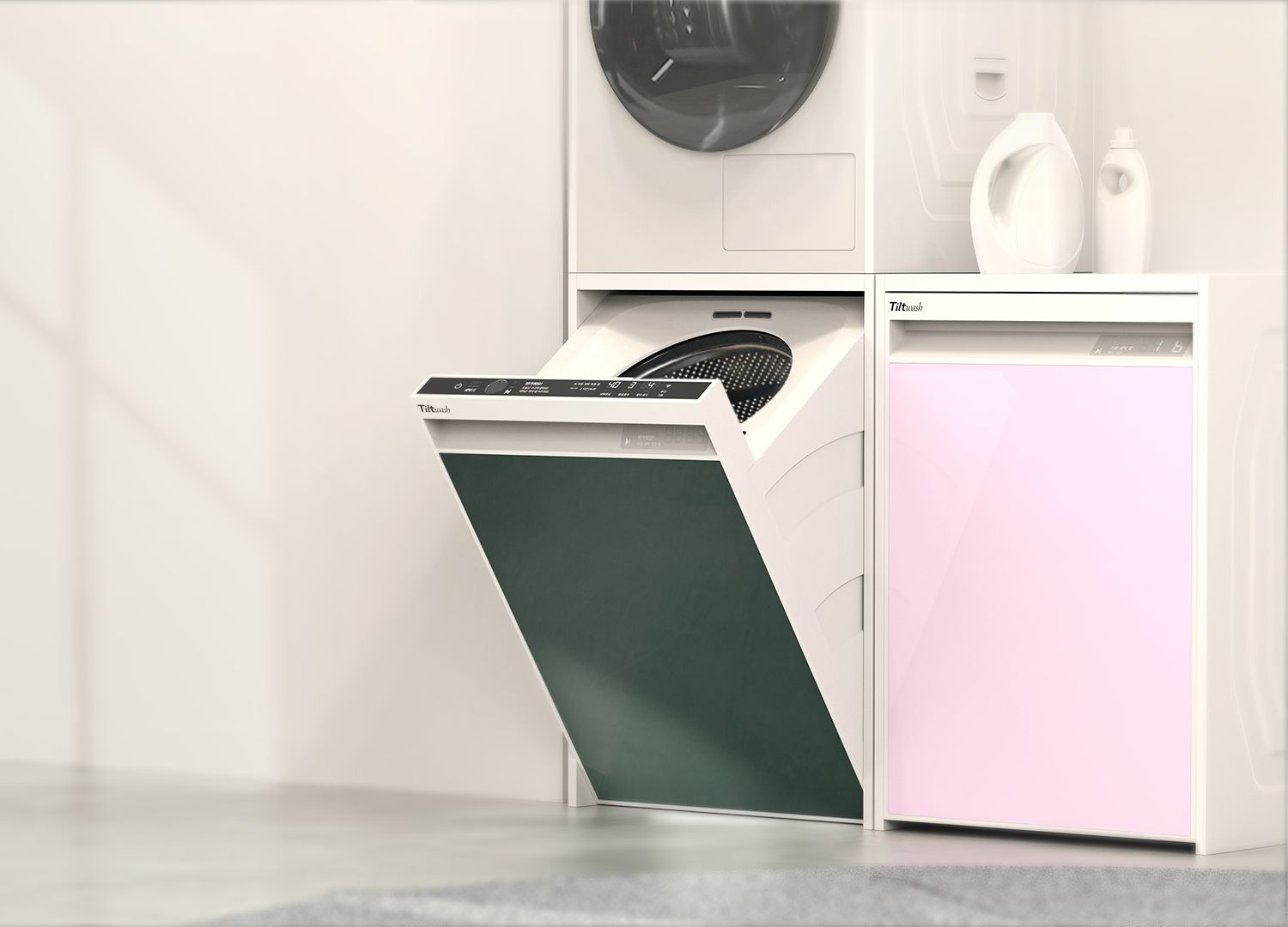The photograph depicts a compact washroom setup within a residential apartment or house, featuring an innovative washer-dryer combination unit integrated into a sleek, white cabinet wall. The washer, located at the bottom, has a distinctive green panel and is designed to fold outward, rotating on a bottom hinge to expose its tumbler for easy loading. Directly above the washer is a dryer equipped with a clear, tinted plastic door—presumably for viewing the contents—which is also adorned with a green control panel.

To the right of this setup is an additional unit with a pink panel, which appears identical to the washer-dryer combination in terms of design and brand, though its specific function remains unclear. On top of this pink unit are white bottles, likely containing laundry detergent and fabric softener. The room's decor includes clean white walls and a modern gray linoleum floor, enhancing the streamlined and functional aesthetic of the space.